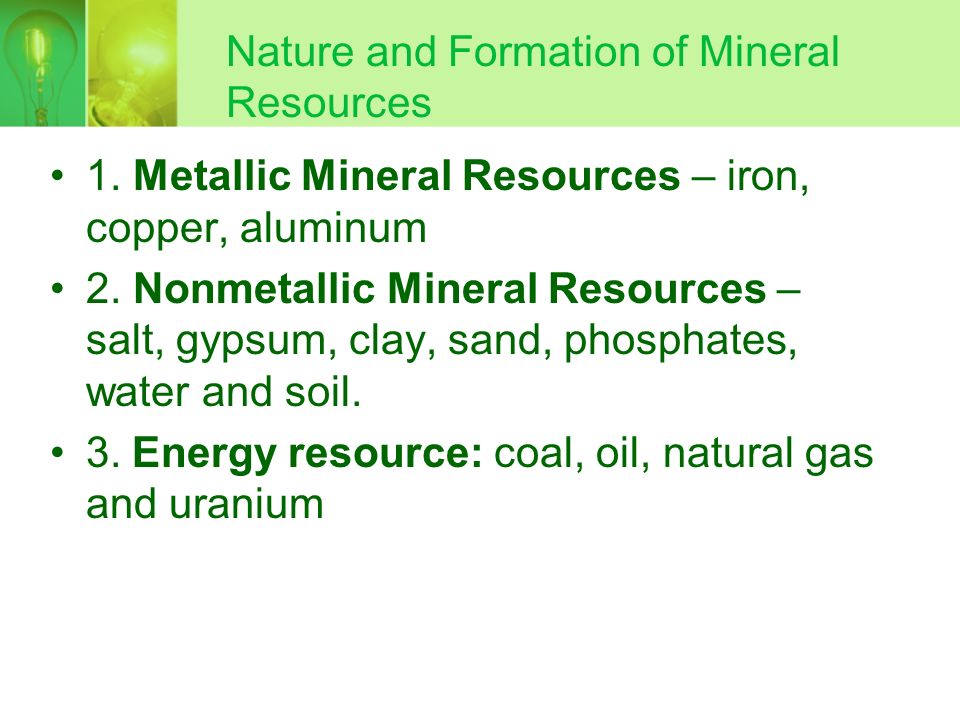The image resembles a slide from an educational presentation, likely formatted in a PowerPoint or similar style, focusing on the nature and formation of mineral resources. It features two small light bulb icons positioned in the top left corner, side by side. The headline, "Nature and Formation of Mineral Resources," is prominently displayed to the right of the light bulbs in a green color against a lighter green background. Below the headline, a detailed list of mineral resources is presented in darker green text with a white background. The list is categorized into three main groups: 1) Metallic Mineral Resources including iron, copper, and aluminum; 2) Non-Metallic Mineral Resources such as salt, gypsum, clay, sand, phosphates, water, and soil; and 3) Energy Resources comprising coal, oil, natural gas, and uranium. The overall layout is contained within a horizontal rectangle, exuding an educational and informative ambiance typical of presentation slides.